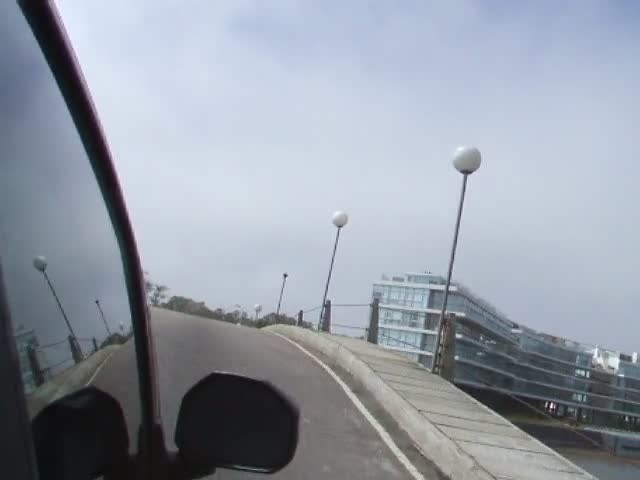This photo, likely taken from the back passenger window of a car, presents an intriguing urban scene that suggests a location outside of North America. The car's unusual octagonal or hexagonal side mirror captures part of the paved road with a full white line to the right, leading to a concrete sidewalk. Along the sidewalk stand tall, stainless steel light poles with retro 70s-style white globe fixtures on top. Toward the right, the sidewalk descends to an area with several stories of apartment buildings—appearing either four or five stories high, potentially including a basement—constructed mostly of glass. The building's modern, slightly curved silhouette features numerous windows and a roof adorned with various elements. Reflecting from the car’s window, faint images indicate the car is moving ahead on a road that slopes slightly, flanked by glimpses of treetops under a light blue and white sky.